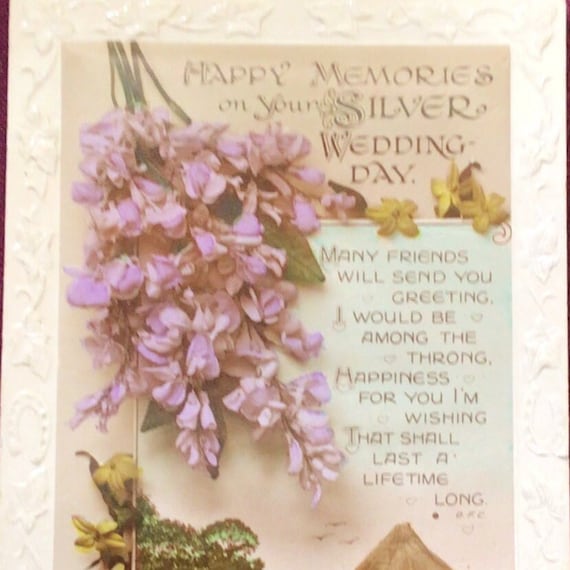This image depicts a detailed photograph of a sentimental greeting card commemorating a silver wedding anniversary. The card is laid flat on a surface adorned with embossed floral designs and a horseshoe motif. The card features an old-fashioned, elegant font that reads, "Happy memories on your silver wedding day. Many friends will send you greeting. I would be among the throng. Happiness for you I'm wishing that shall last a lifetime long." Surrounding the heartfelt message, a spray of beautiful flowers adds a touch of color: purplish-pink blooms cascade from the top left, while additional yellow flowers with green stems embellish the bottom left. A small cluster of yellow flowers is intertwined within the text at the top right. The background of the card boasts a soft, peach-brown hue, enhancing its vintage charm. No people or animals are visible in the image, and there are no watermarks or signatures present.